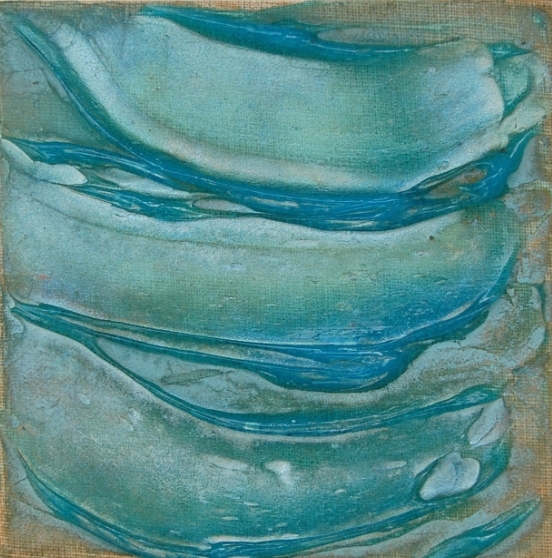This photograph captures an up-close view of a square canvas or natural linen surface, measuring approximately five inches by five inches. The canvas is adorned with a unique, heavily textured application of paint, which includes three prominent swipes. The color palette features a lighter pearlescent white, blended with a homemade mixture of turquoise blue and shimmery sage green. The paint is unevenly mixed, creating a rich, textural contrast that reveals various subtleties in color. The pearlescent sheen enhances the depth, allowing glimpses of the original linen material to show through. Notably, the painted swipes form a pattern resembling a large, stylized "E" shape, which is bordered by darker lines and set against a background that hints at both the original canvas and a touch of grey. There is no text, signature, or date visible on the artwork.